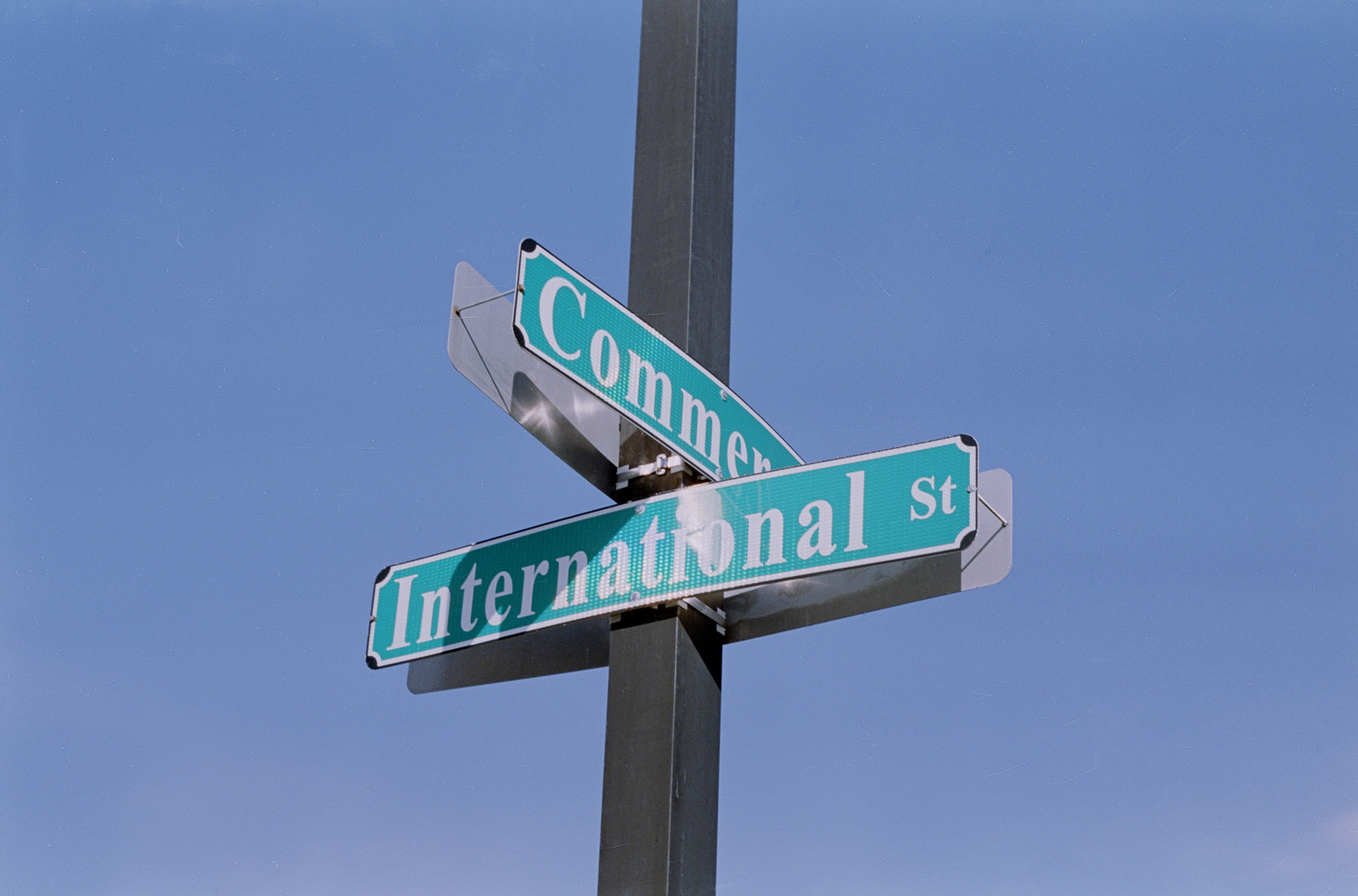The image depicts a first-person POV close-up of a tall, square, black metal pole with two street signs attached, captured at a slight upward angle against a clear blue sky. The lower sign, positioned horizontally, reads "International Street" in bold white letters on a green background with a white border. Above it, another sign mounted at a 90-degree angle displays "Commerce" in white letters on a green background, although only "C-O-M-M-E-R" is fully visible. Both signs are duplicated on the opposite side of the pole for visibility from both directions, although we can only see one side of each sign in this photograph. The pole is centered in the image, with equal lengths of the pole extending above and below the signs.